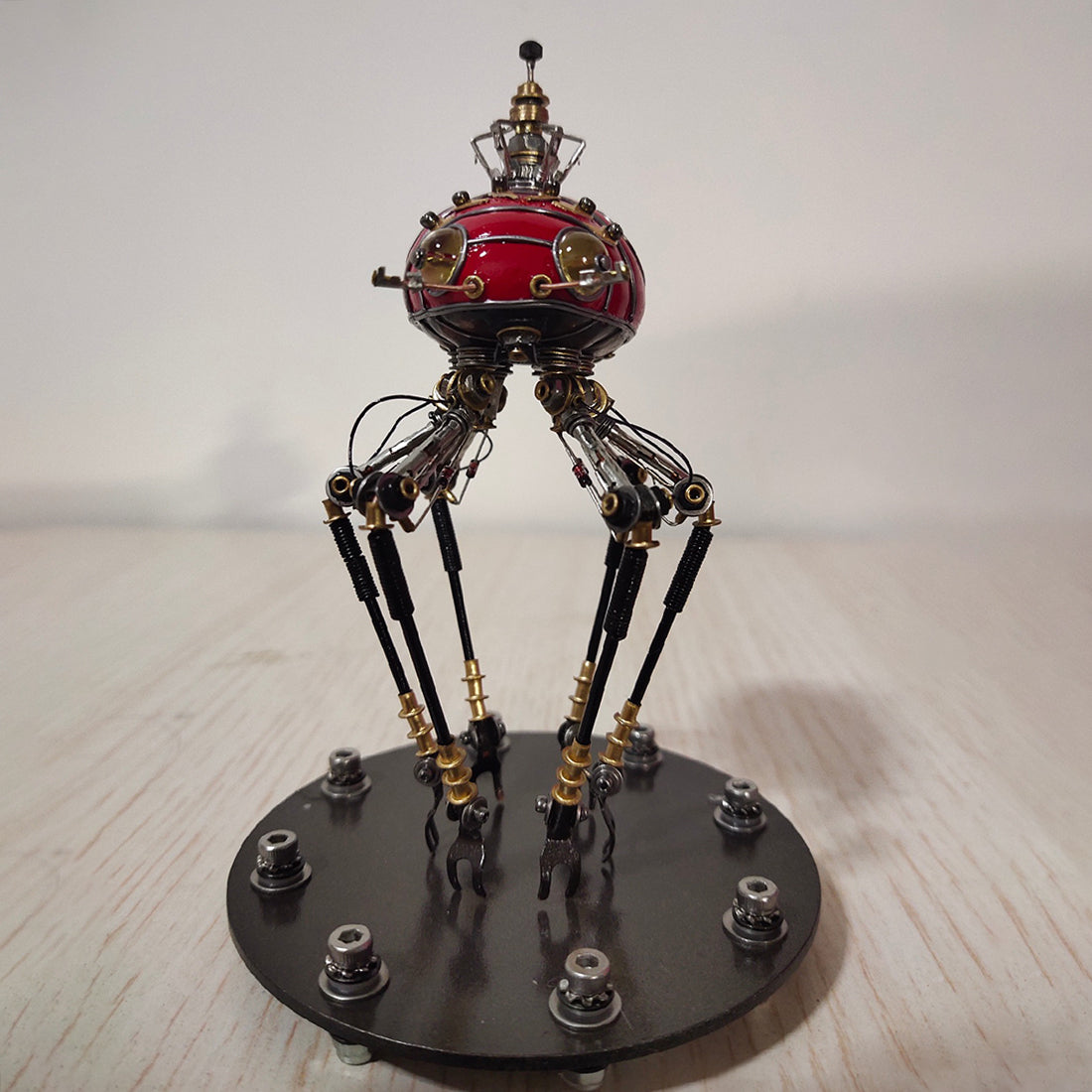The image depicts a steampunk-inspired metallic object resembling a robotic insect or octopus with six articulated legs. The body of the device is a red, egg-shaped dome, with two glass-like eyes and an antenna-like appendage on top, enhancing its otherworldly appearance. The legs, festooned with pulleys, wires, and gears, emerge symmetrically from a round circular metallic base. This base, which rests on a white wooden table against a gray and black backdrop, is adorned with eight bolts around its edges. The intricate design features bronze or gold detailing encircling the red dome, and a turret-like structure extends from its apex, crowned with a small black point and circle. The overall impression is of a meticulously crafted, multi-legged contraption poised in a static yet dynamic pose, merging art and mechanical wonder.